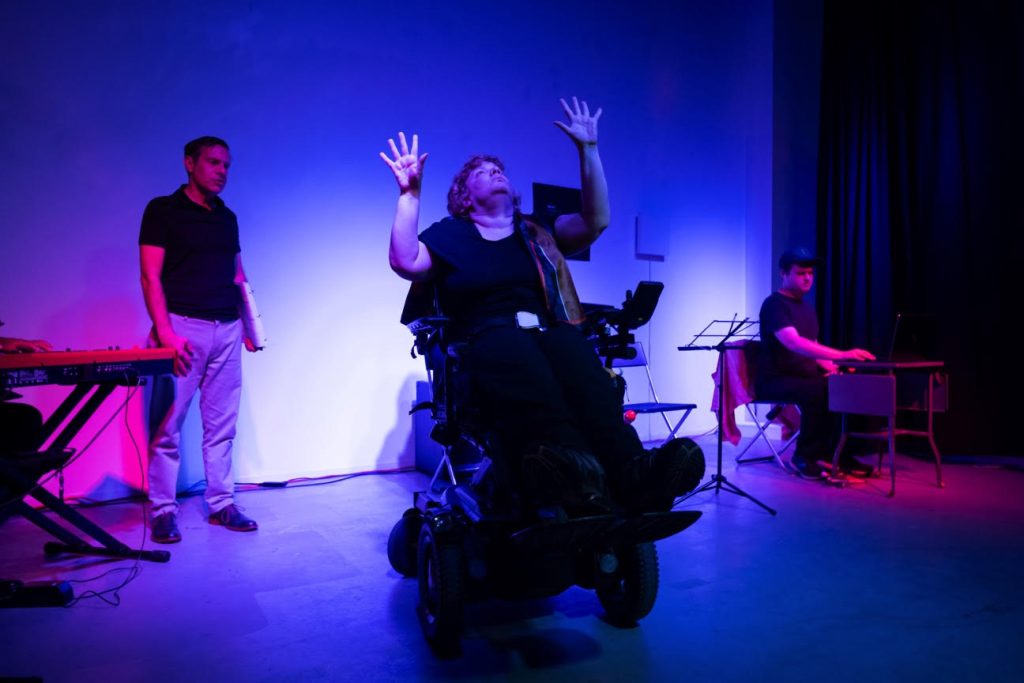The image depicts a detailed scene of a stage performance bathed in blue light. Center stage is an elderly woman of larger stature, seated in a mechanical, motorized wheelchair with adjustable height. She is looking upward with her head tilted back, and her arms raised, fingers spread wide. She wears black clothes and appears to be secured to the chair with a waist band. To her left stands a man in a black T-shirt, grey pants, and black shoes, holding papers in one hand. On the left side of the stage, a person is seated playing an electric keyboard attached with wires. On the right side, another man is seated at a small black table, which may be a desk or keyboard. The background features a screen illuminated with blue, white, and pink lights. Further right, a black screen and various stage props, including a chair and a stand with a blank paper platform, can be seen. Additionally, there is a white wall with a meter box and other fixtures. The overall ambiance of the stage is serene, emphasized by the blue lighting, although not a spotlight, contributing to a cohesive and intricate performance setup.